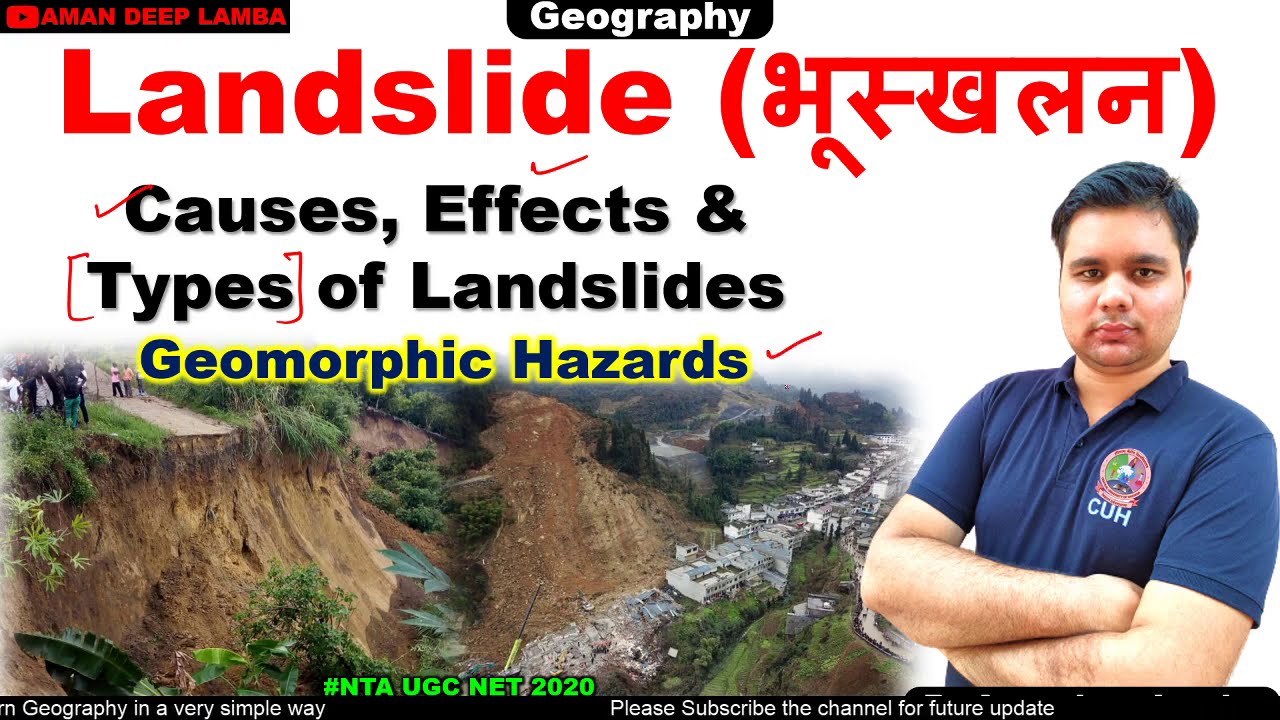The image depicts a YouTube advertisement featuring a man with dark hair wearing a blue polo shirt with “C-U-H” printed on it in white, standing on the right side with his arms crossed and a serious expression. The upper left corner displays “Amman Deep Lamba” alongside the YouTube logo. The central text, bordered in black, reads “Geography” in white font, followed by “Landslide” in red, and “Causes, Effects, and Types of Landslides” in black. Below this, “Geomorphic Hazards” is highlighted in blue and yellow font. The image captures a dramatic landslide scene, showing a road that has collapsed into a dirt-filled chasm surrounded by trees; houses and concrete structures lie in ruins at the base. People stand on the edge of the eroded land, looking down at the destruction. The background provides a stark contrast of natural beauty with distant trees and the devastation caused by the landslide. This advertisement encourages viewers to subscribe for more geography content, including NTA UGC NET 2020 topics.